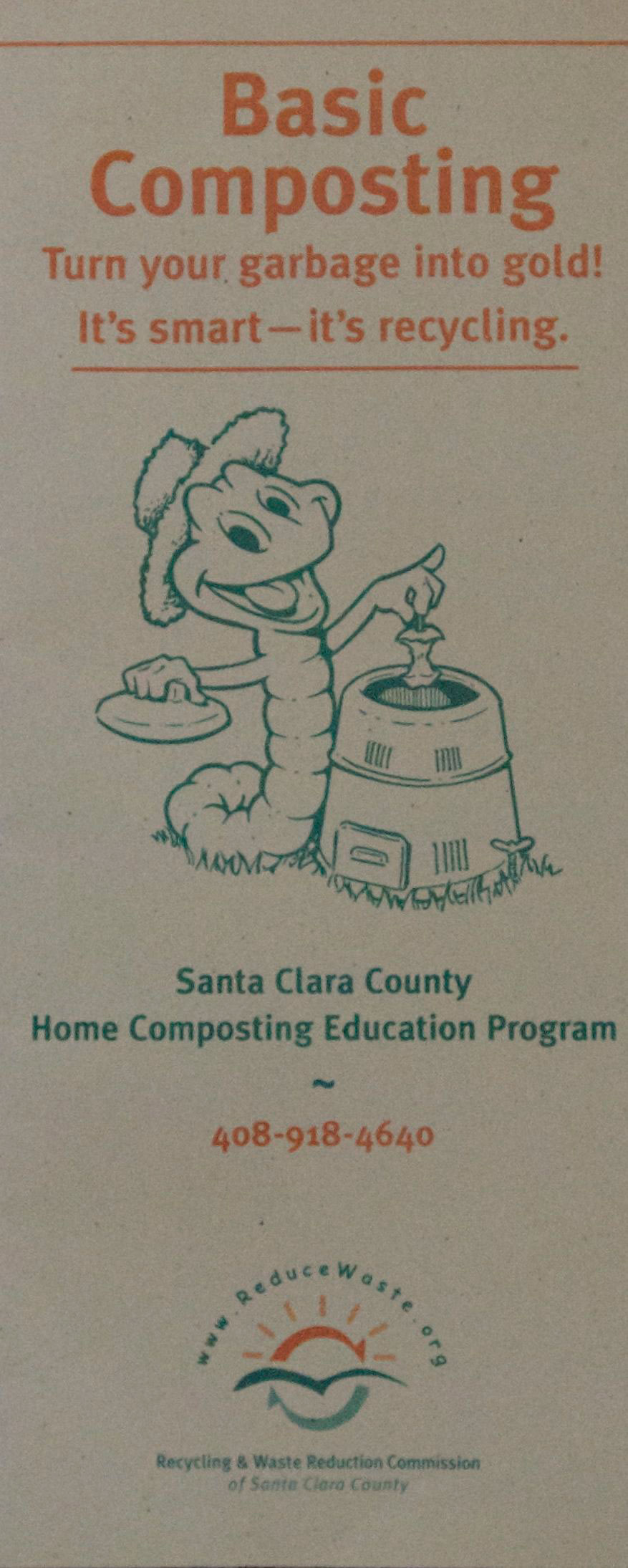The image is a tall, vertical pamphlet on composting with a gray background. At the very top, an orange bar spans the width of the leaflet, beneath which the heading "Basic Composting" is displayed in large, gray text. Directly below, in slightly smaller orange text, it reads "Turn your garbage into gold. It's smart. It's recycling." This is also framed by an orange bar underneath. Beneath this section, there is a detailed drawing of a cheerful green worm wearing a hat, holding an apple core aloft in one hand while lifting the lid of a cylindrical compost bin with the other hand. Below the illustration, in green text, it states "Santa Clara County Home Composting Education Program." Further down, there is a contact number in orange: 408-918-4640. A website address, www.reducewaste.org, is printed in an arch shape beneath the contact number. At the bottom, an emblem features orange lines and a blue outline of bird wings above a light green semicircle. The very bottom of the pamphlet, in small green text, reads "Recycling and Waste Reduction Commission of Santa Clara County."